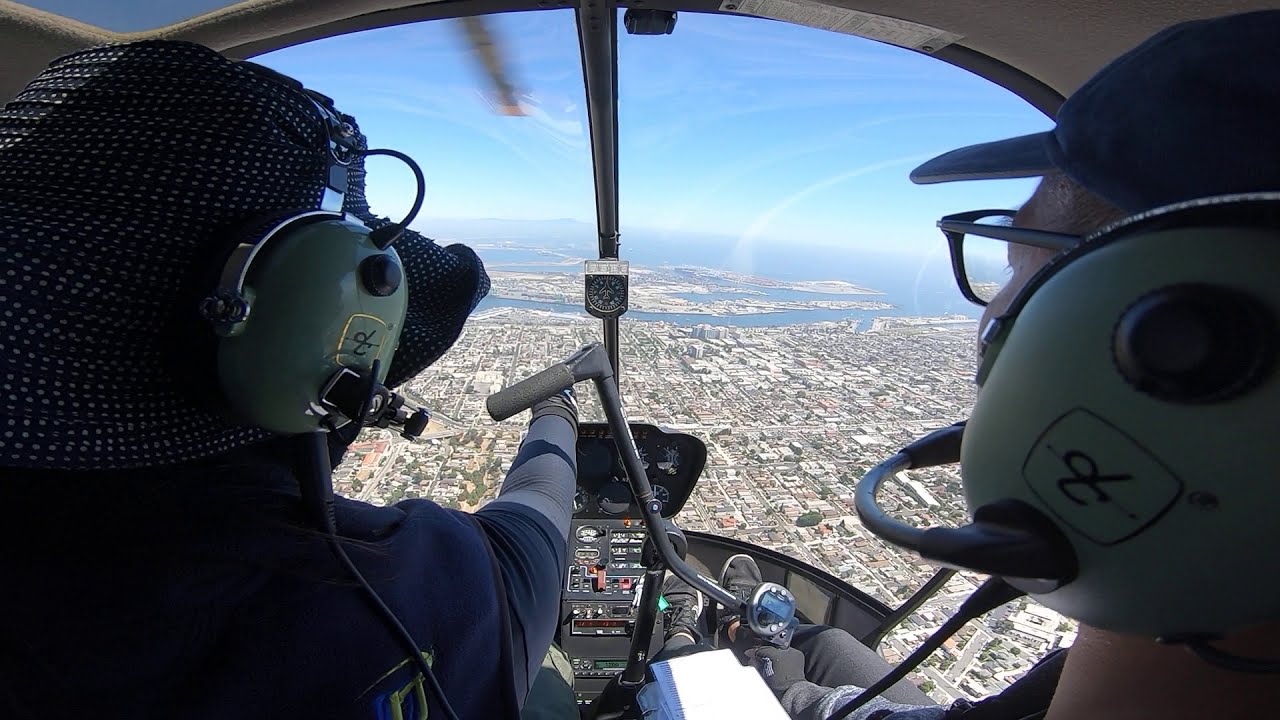This photograph captures the interior of a helicopter, showcasing a pilot and a co-pilot or possibly a passenger, as they fly over a densely populated metropolitan area. The wide-angle or fisheye lens used makes the windshield appear extensively large, highlighted by the blurry presence of one of the helicopter's whirring blades visible at the edge of the frame. The two people, both seemingly men, are viewed from behind. One is dressed in a blue shirt and a blue and white bucket hat, while the other wears a blue baseball cap. They both have light green headphones on, presumably for communication. Below them, the sprawling cityscape is clearly visible, and in the far distance, there is a body of water, possibly a river or lake, with additional landmasses seen even further beyond. The interior of the helicopter reveals parts of the control panel between their seats, including what might be an altimeter, and the feet of the two individuals.